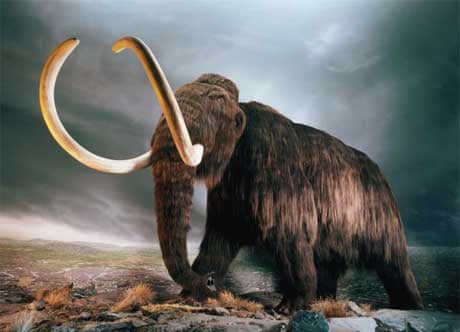This painting features a lifelike representation of a woolly mammoth, an extinct species related to elephants. The mammoth is depicted with long, shaggy brown fur and massive, curved ivory tusks that form a wide arch, standing in profile view with its head slightly turned towards the viewer. One side of its body is illuminated by light from the right, revealing a lighter tan patch on its otherwise dark fur. The tusks are lighter, cream-colored, contrasting with the mammoth's darker fur. The backdrop portrays a dramatic and stormy landscape, with a dark, cloudy sky suggesting an approaching storm. The mammoth stands on uneven, rocky ground with sparse vegetation, including short green, orange, and brown weeds, indicative of a harsh, tundra-like environment typical of the Ice Ages.